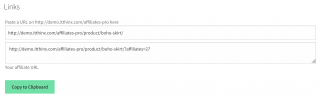This image is notably small, approximately an inch by two inches in size, necessitating browser maximization for minimal readability. At the very top, the word "Links" is displayed. Below it, in extremely tiny and slightly blurry lettering, appears the instruction "Paste a link" or "Paste a URL," albeit the exact text is indiscernible due to its minuscule size and clarity. Beneath this text are two white horizontal rectangular boxes with illegible text due to their small font. Further below, there is additional text without any bordering. At the bottom of the image, surrounded by a green border, are the words "Copy to clipboard." The lower text box features an interactive area meant for enlarging the text or expanding the box to accommodate more content. The entire image is challenging to view clearly without zooming in significantly.